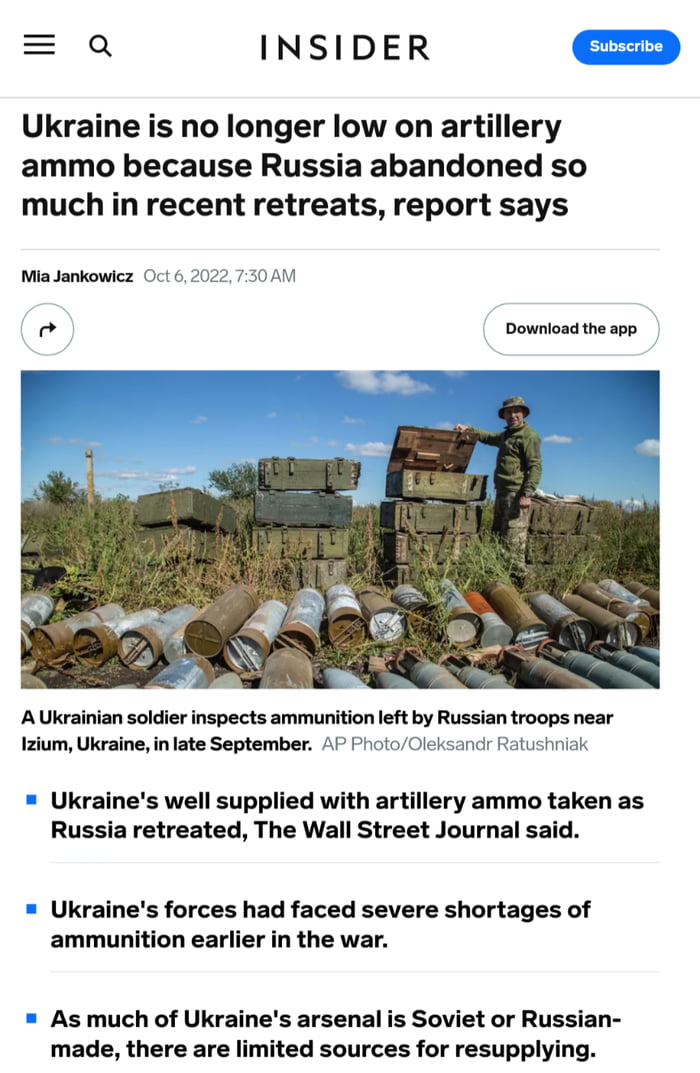This is a detailed screenshot of an article from Insider, prominently displayed with the website's name at the top center. The interface includes a burger menu icon on the top left, followed by a magnifying glass for search functionalities. On the top right, there is a blue 'Subscribe' button for users to join the newsletter and receive the latest updates. Just below, there's a mention that users can download the Insider app.

The article is titled, "Ukraine is no longer low on artillery ammo because Russia abandoned so much in recent retreats, report says." It is authored by Mia Jankowicz and was published on October 6, 2022, at 7:30 a.m. Accompanying the article is a photograph featuring a Ukrainian soldier inspecting large, green and blue suitcases filled with ammunition left behind by Russian troops near Izium, Ukraine. The top left corner also includes icons likely for sharing the article or returning to the previous page.